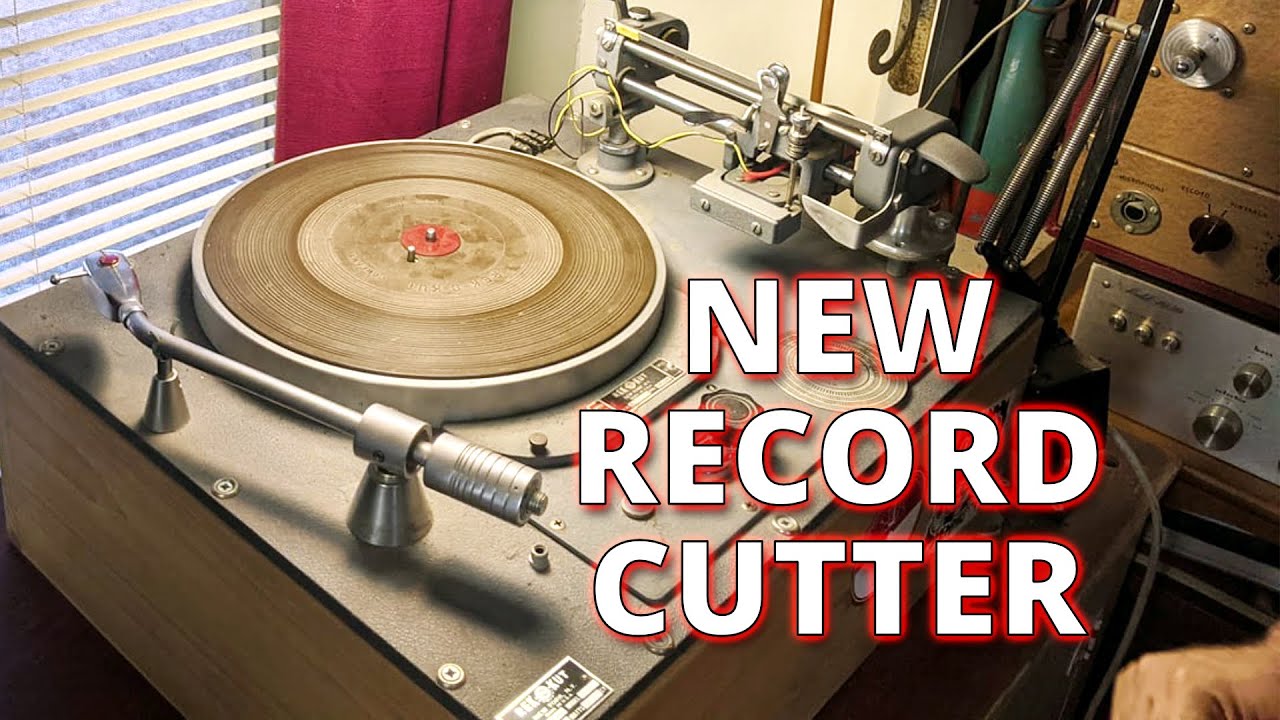The photograph showcases a vintage record cutter situated in a domestic setting, likely someone's home. The record cutter features a rectangular design with wooden sides and a black top secured by screws. A silver, stainless steel arm extends towards a black record, indicating its function. The cutter is adorned with metallic parts and sections with golden and orange hues. The image has been edited to include text that reads "New Record Cutter" in white, superimposed on a red background, prominently positioned at the bottom right, reminiscent of a YouTube thumbnail. Behind the record cutter, there are window blinds and a red curtain, with cream-colored walls partially visible. To the right of the cutter, additional audio equipment with various knobs and input options is present, all resting on a brown surface.